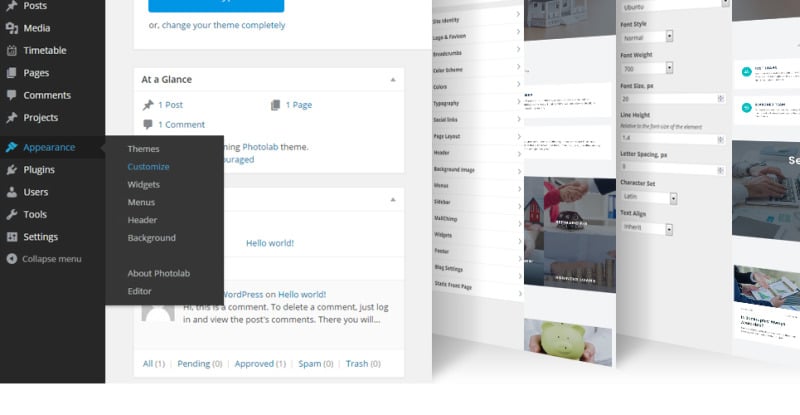The image is a screenshot of a web page interface, likely a content management system dashboard. On the left-hand side, there is a vertical black column featuring menu tabs, each accompanied by an icon. These tabs include: Posts (represented by a thumbtack icon), Media (with a painting palette icon), Timetable (displaying a calendar icon), Pages (shown as stacked paper icons), Comments, Projects, Appearance, Plugins, Users, Tools, Settings, and a Collapse Menu option.

To the right of this column, the main section of the page showcases a large header that reads, "Or Change Your Theme Completely." Below this header, there's a prominent blue rectangular box. Further down, an "At a Glance" section summarizes the site's content, indicating there is one post, one comment, and one page.

In addition, a segment below titled "Hello World!" introduces the first post. To the far right, the image depicts three other pages displayed in a slightly three-dimensional view, tilted to the right, giving the appearance of layered, overlapping documents. This detailed arrangement provides a comprehensive view of the web page's layout and functional elements.